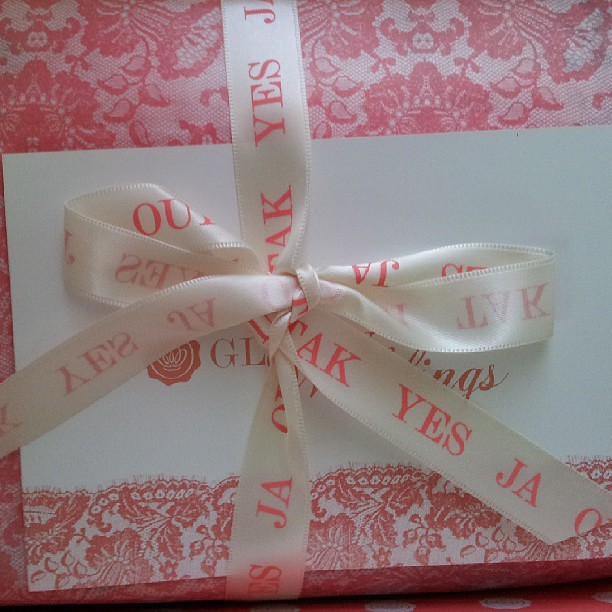The square image depicts a beautifully wrapped gift box adorned with a pink and white floral pattern that resembles lace. A white envelope with some embossed writing rests on top of the box, partially visible. Both the gift box and the envelope are elegantly tied together with a white ribbon featuring pink inscriptions of the word "yes" in various languages, including "ja" and "tak." The sides of the package reveal a darker shade of pink, possibly due to lighting, and the ribbon is hand-tied into a large bow. The lower right corner of the image hints at a surface with pink and white polka dots.